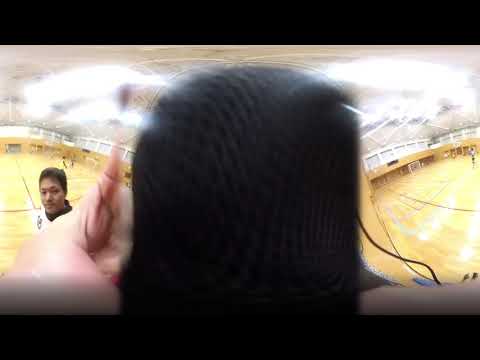This horizontally aligned, smaller-sized image is notably blurry and encased by thick black borders at both the top and bottom, resembling a video capture. The central portion of the photo appears distorted and warped, almost as if a panoramic image has been flattened. Dominating the center is a large, black textured object reminiscent of the head of a giant microphone, obscuring much of the image's middle. On either side of this central object, the scene depicts what seems to be an indoor sports arena or gym with a yellowish hardwood floor marked with black lines resembling playing field boundaries. Bright white lights illuminate the ceiling above. To the left, a man with short black hair, dark skin, and wearing a white top over a high-necked black shirt stands with his hand raised towards the camera or microphone-like object. In the lower left part of the image, another figure, also a man, wearing a black and white shirt, can be faintly seen. In the distance on the right side of the image, more figures and the same style of gym floor are observed, suggesting either another view of the same gym or a similar, nearby location.